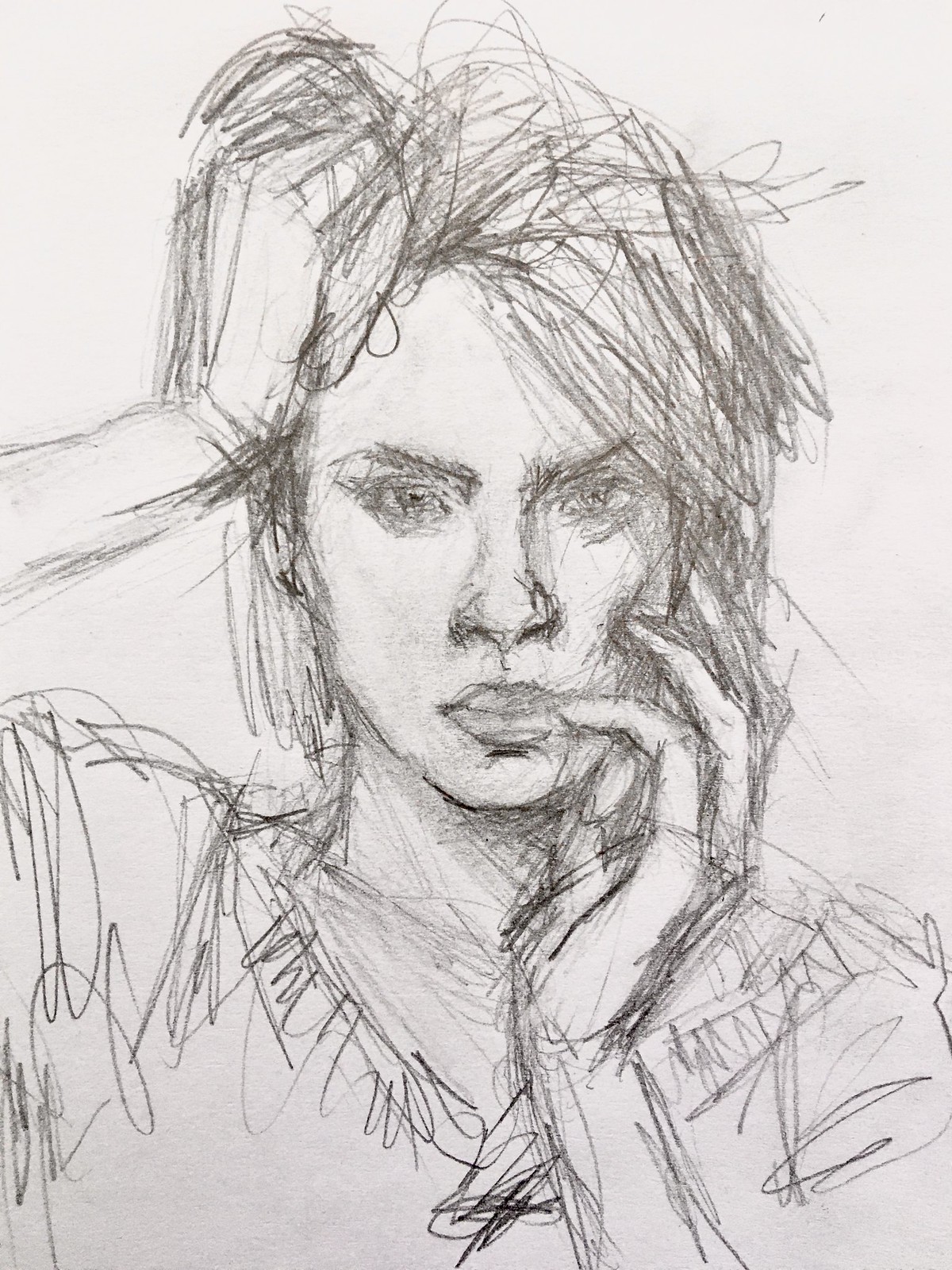This captivating pencil or charcoal drawing portrays a young woman rendered entirely in grayscale, set against a light gray background. Her chin-length hair, slightly messy and puffy at the top, falls straight with several strands sticking out. With her right hand, she tousles her hair on the right side of her head. Her gaze is direct, her expression serious, characterized by full lips, fair skin, almond-shaped eyes, and eyebrows that taper towards the nose and rise towards the outer edges. She has a conventionally shaped nose. Her left hand is held up to the left side of her face, with her thumb resting under her chin and three fingers splayed along her cheek. The woman wears a blouse with a scoop neck, depicted with minimal detail through loose, scribbled lines.